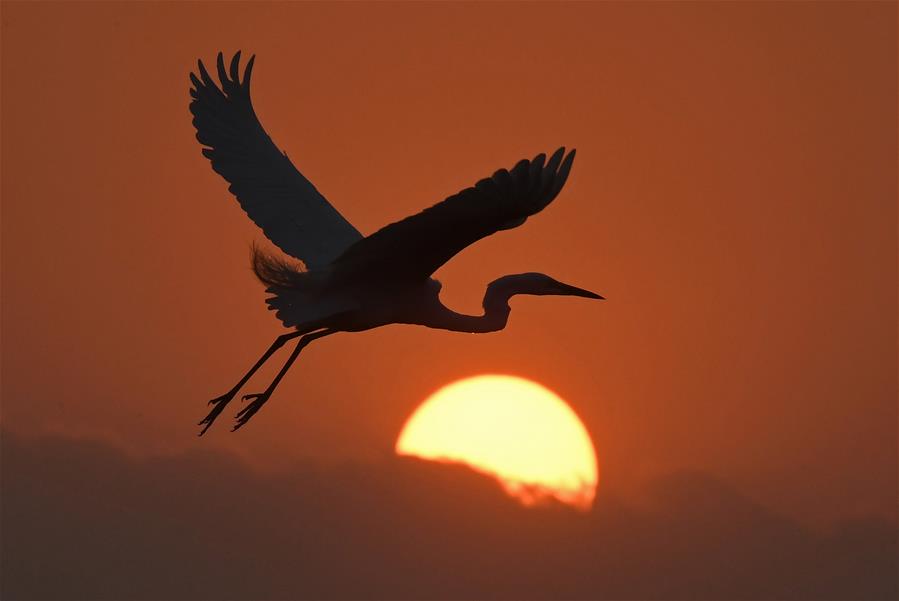The image captures a breathtaking scene of a sunrise or sunset with the sky painted in vivid orange and rusty tones. At the center of this spectacular display is the sun, a glowing yellow orb partially obscured by thick, darker orange clouds. Just to the left of the sun, a large bird—most likely a stork or crane—is captured in elegant flight. The bird is rendered in a striking black silhouette, its long neck and beak pointing forward. Its wings are fully outstretched and raised high above its head, while its legs trail straight out behind it. This compelling composition showcases a harmonious blend of natural elements, focusing primarily on the silhouetted bird set against the brilliant, warm-hued backdrop.